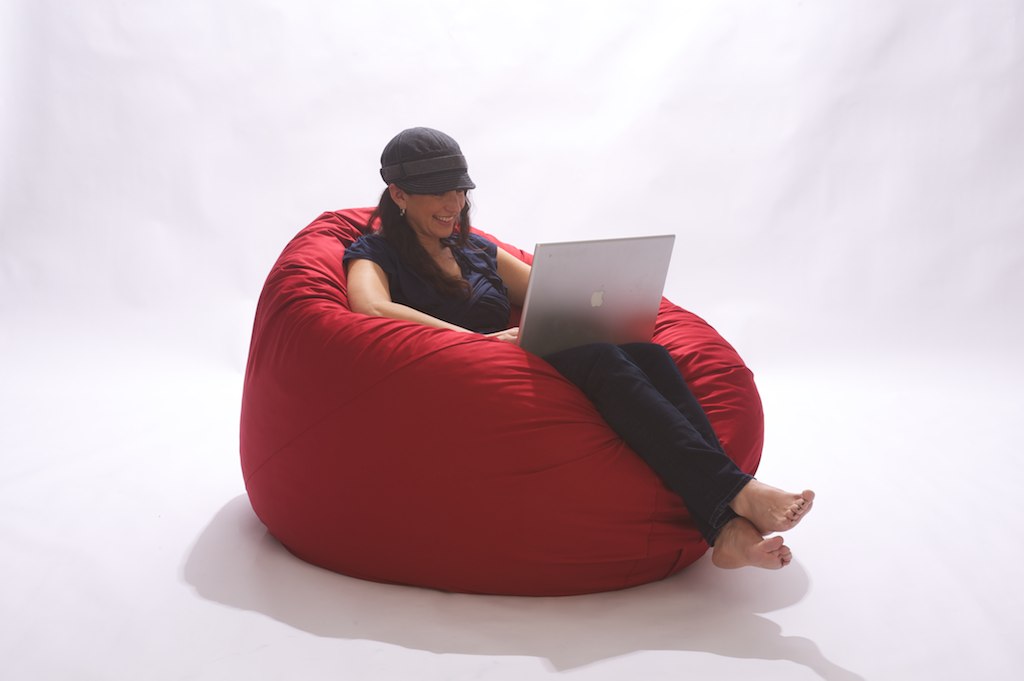In this image, a barefoot Caucasian woman is seen sitting comfortably in a large, round red beanbag chair, giving the impression of being slightly sunk into it, with only her legs, arms, and head visible. She's dressed entirely in dark colors, wearing a black cap, a dark blue v-neck top with short sleeves, and black jeans. Her longish hair peeks out slightly from beneath her cap. The woman is smiling as she types on a silver Apple MacBook, which rests on her lap, and her toenails are painted red. She wears hoop earrings, visible particularly in her right ear. The bright, blurry white and gray background casts a pronounced shadow beneath the beanbag chair and her feet, almost giving the illusion she's sitting on a cloud.